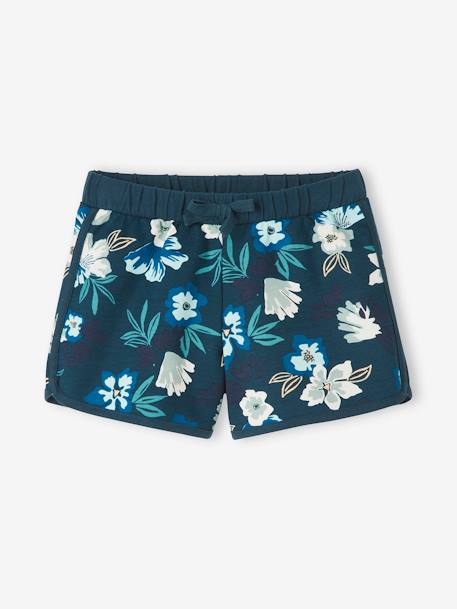The image features a pair of dark blue swim trunks adorned with a floral pattern consisting of varying shades of blue and white flower petals. The shorts are laid flat on a white background, displaying a top-down view. They include a dark blue elastic waistband and a blue string tie positioned at the center of the waistband, typical of swim trunks. The background provides no additional context, leaving the size and intended wearer—whether a child or an adult, male or female—ambiguous.